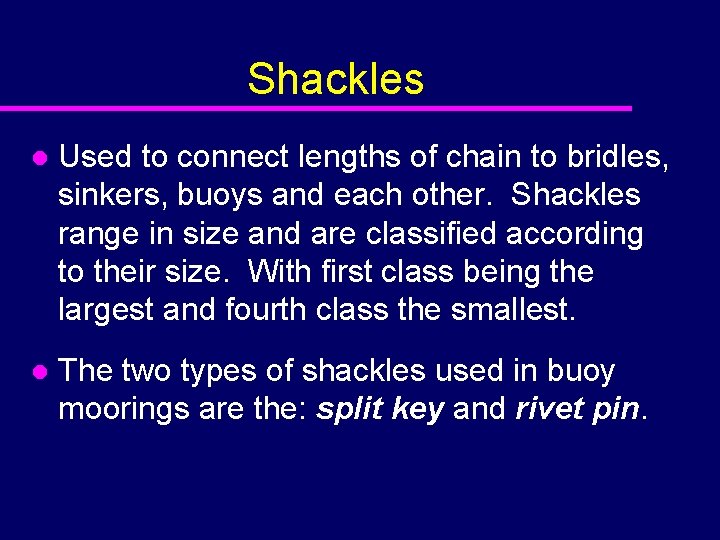This detailed presentation slide features a bold, dark blue background with a distinct, bright yellow title centered at the top that reads "Shackles," emphasized by a pinkish-purple line below it. The slide is well-organized and contains no images, focusing solely on textual information. The text is written in a mix of upper and lowercase letters in white for readability against the dark background. 

The content is structured into two purple bullet points, effectively spaced to maintain clarity. The first bullet point states: "Used to connect lengths of chain to bridles, sinkers, buoys, and each other. Shackles range in size and are classified according to their size, with first class being the largest and fourth class being the smallest." The second bullet point informs: "The two types of shackles used in buoy moorings are the split key and the rivet pin."

Overall, the slide appears to be a clean, traditional information presentation, possibly created using PowerPoint, with the text centrally aligned and clear labels for easy reading.